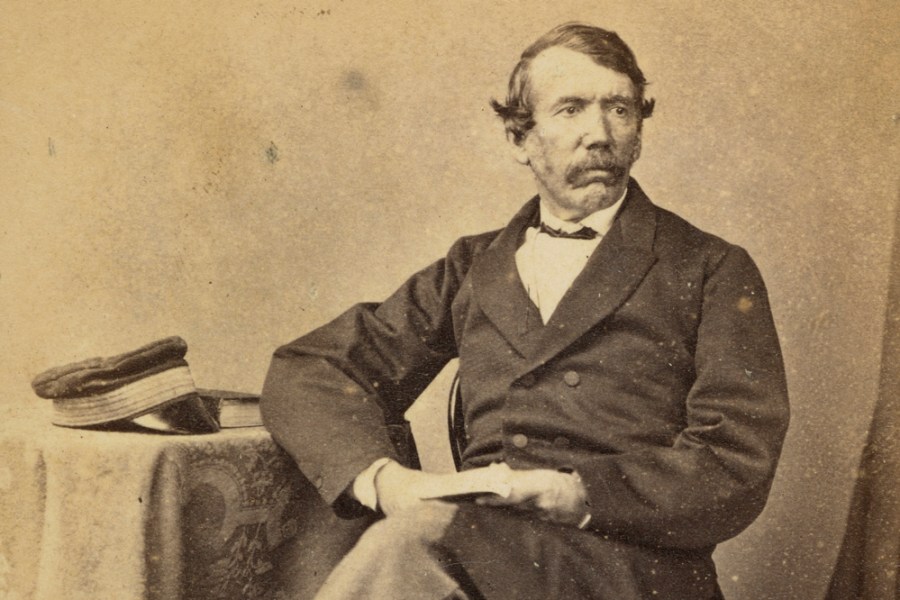This sepia-toned, grainy photograph, likely from the mid-19th century, captures a distinguished, middle-aged gentleman with dark, straight hair and a bushy mustache, meticulously combed downward. He is dressed in a dark, double-breasted suit with a collared white shirt and a bow tie, and his gray trousers are visible as he sits with his legs crossed. The man, who looks serious and contemplative, props his right elbow on a lace-topped end table beside him, slightly turned to the right. In his hands, he holds a book while another book is placed on the table. Also on the table is a black hat with a lighter-colored trim and stripes. The photograph is speckled with spots, adding to its aged appearance.